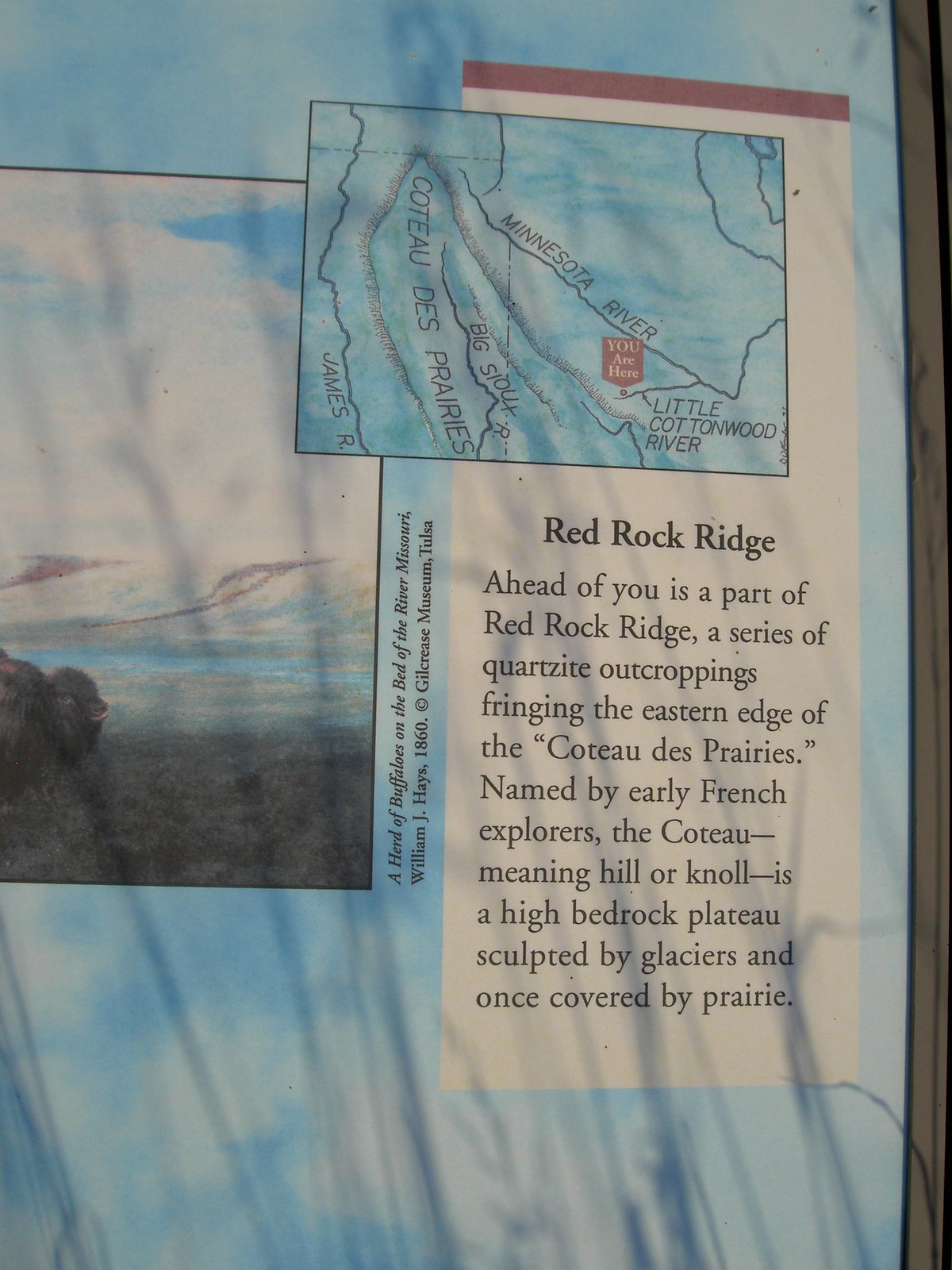This photograph captures an informational display likely found in a museum or park, describing historical and geographical details about the region. The backdrop of the display is light blue, featuring a predominant map at the top marked with labeled areas and rivers, including the Minnesota River and the Little Cottonwood River, both delineated in black lines on a blue map. Below this map, encased in a white rectangular text box, the following information is presented: "Red Rock Ridge. Ahead of you is a part of Red Rock Ridge, a series of quartzite outcroppings fringing the eastern edge of the Coteau des Prairies. Named by early French explorers, the Coteau, meaning hill or knoll, is a high bedrock plateau sculpted by glaciers and once covered by prairie."

Adjacent to the text and map on the left side, there is an image of a buffalo or bison, albeit partially visible. This image features shades of blue, white, and brown, likely depicting a scenic view of the sky and ground. The accompanying caption of the buffalo image reads: "I heard of buffalo on the bed of the river, Missouri, William J. Hayes, 1860 copyright, Gilcrease Museum, Tulsa." The display also includes a brown border on the right side, consolidating its detailed presentation.